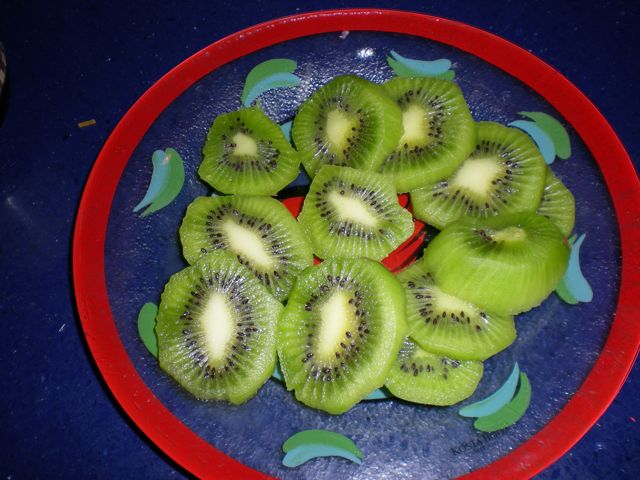In this close-up photo, we see a striking arrangement of twelve sliced kiwis displayed on a blue plate with a red rim. The plate features a repeating pattern of U-shaped green and blue designs, which add an extra layer of visual interest. The kiwis, peeled to reveal their vibrant green flesh, are sliced in varying thicknesses, from extremely thin to about an inch. They are meticulously arrayed in a semi-circular pattern, allowing glimpses of the plate's design and hints of a mysterious red image beneath them, possibly a flower. Light from a camera flash adds a reflective shine to the scene. The overall presentation, set against a dark blue background, highlights the contrasting colors and shapes, making the image both visually captivating and detailed.